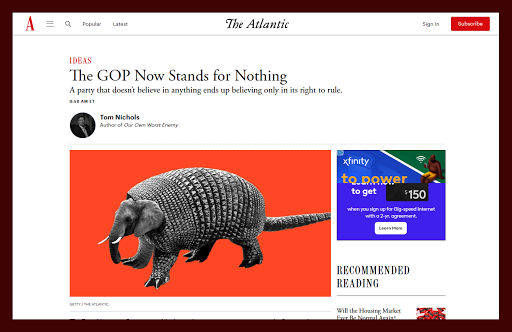This is a detailed, edited screenshot of The Atlantic's website. The Atlantic, an esteemed journalism outlet akin to an online magazine, features a clean layout with a predominantly white background at the top. Centered on this white backdrop, "The Atlantic" is prominently displayed. To the right, a large red "Subscribe" button catches the eye, and to its left, "Sign In" is inscribed in small black letters in the far-left corner.

On the top-left corner, a capital red "A" symbolizes The Atlantic. Adjacent to the "A" is a menu icon, while to its right, a magnifying glass icon signifies the search function. Nearby, the headings "Popular" and "Latest" are written in small black letters.

Below this header, "Ideas" is highlighted in bold red letters in the top-left section. Beneath it, a striking headline in large black letters declares, "The GOP Now Stands for Nothing." This is followed by a subheading in black text: "A party that doesn't believe in anything ends up believing only in its right to rule."

To the left of this text, the author's profile picture is displayed in a circular format. Below the photo, it indicates that the author has penned a book. The most visually arresting element on the page is a large image below the text, featuring an armadillo with the head of an elephant, set against an orange background.